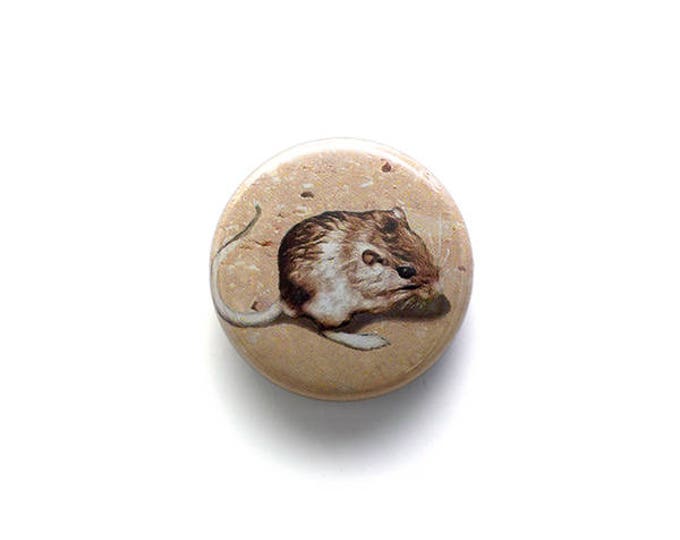The image depicts a circular, glossy button, likely found at a gift shop or zoo, set against a white background with a slight shadow beneath it. In the center of the button, there's an illustration of a small brown rodent, possibly a hamster or mouse. The creature has distinct black eyes, white and brown fur, and a white belly and feet. It appears to be standing with its front paws positioned near its mouth, as if eating. The animal's tail, which is gray and curls upward in a C-shape, extends towards the left. The button itself is a beige or tan color, and the ground depicted beneath the rodent features fine cracks resembling a hard or dirt surface. The overall scene is detailed with careful attention to the tiny animal’s features and the textured background.